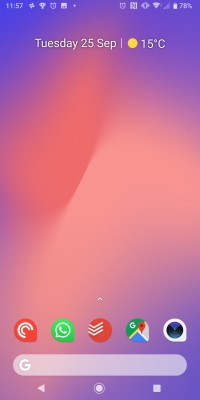Vertical smartphone screenshot featuring a softly gradient background transitioning from light baby pink at the center to a blend of darker pink, purple, and blue towards the edges. At the very top of the screen, the status bar displays the time as 11:57 a.m., flanked by various icons including a trophy and a folder on the left, with the Wi-Fi, signal, and battery (at 78% capacity) icons on the right. Also present in this bar is information indicating it’s Tuesday, the 25th of September, and a weather update showing a sun icon with a temperature of 15 degrees Celsius.

The bottom section of the screenshot showcases a row of app shortcuts, featuring icons for WhatsApp, a nondescript app, Google Maps, and a camera. Just below this row sits a prominent Google search bar, and at the very bottom, the traditional navigation buttons – back, home, and recent apps – are clearly visible. The overall design of the screenshot is minimalistic and clear, providing easy access to basic functions and essential information.